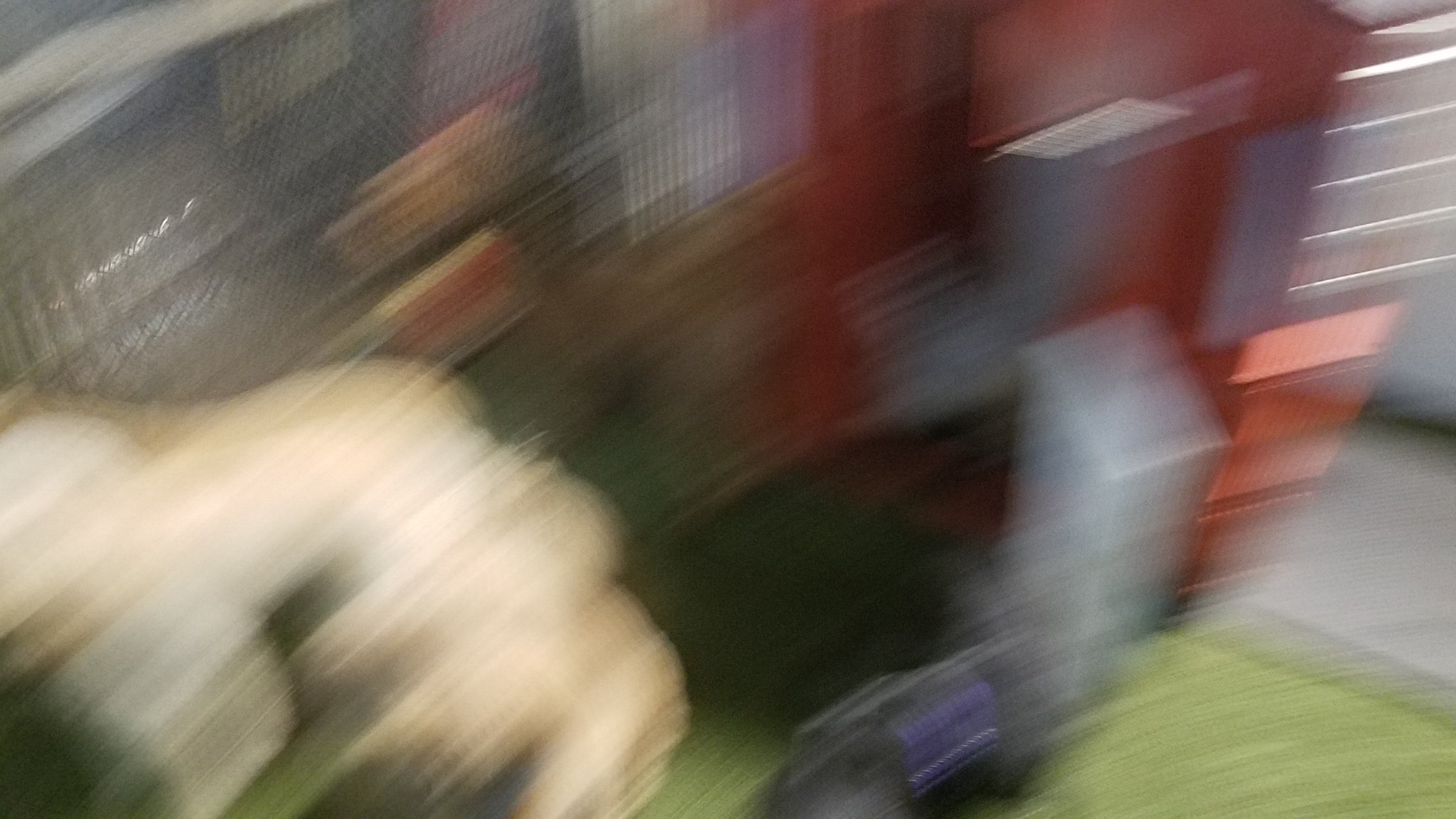This image, captured with a moving camera, showcases a complex scene with various elements. The floor prominently displays a vibrant green color, transitioning to gray concrete at the upper right side. In the bottom-left corner, there is a skin-toned object that appears to be a clenched fist or hand emerging into view. Behind this hand, the background includes a gray element, potentially a wall or structure. Centrally, there's a window bordered by a striking red surface. The red color dominates the middle section, bending slightly and continuing vertically. This red region is framed with gray on the edges, complementing the vibrant hue. Beneath this, a red area resembling aluminum siding is visible. In front of this siding stands a tall, square, gray object, adding a contrasting dimension to the colorful backdrop.